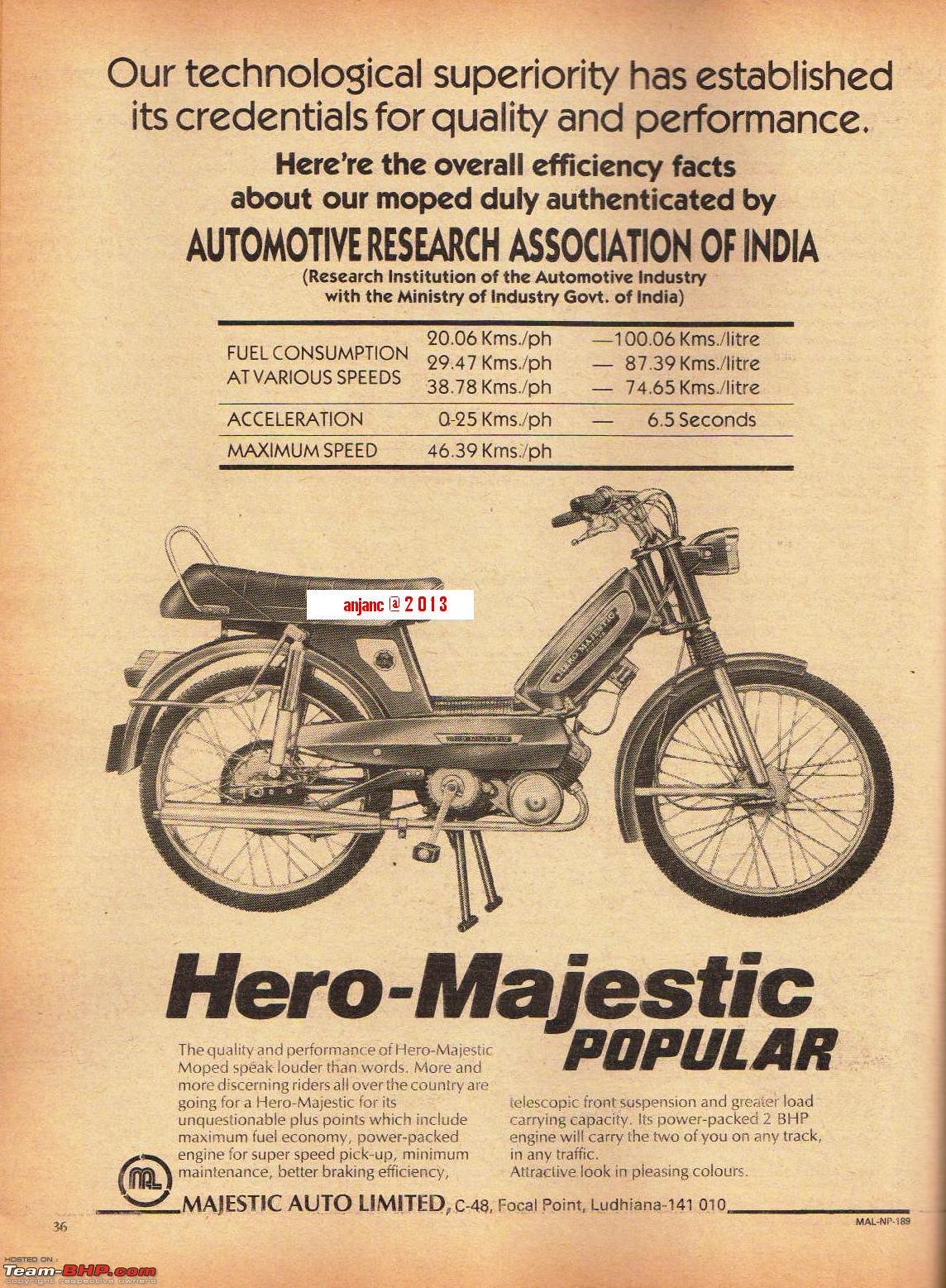The image is a scan of an old, weathered advertisement on discolored, yellowing paper, darker around the edges. It features black writing with lines of text above and below a central picture of a moped, shown from a sideways view. At the top, the bold headline reads, "Our technological security has established its credentials for quality and performance." Below this is a detailed chart with authenticated efficiency facts about the moped, such as fuel consumption, acceleration, and maximum speed, certified by the Automobile Research Association of India. Under the moped image, a prominent label in large font declares, "Hero-Majestic Popular." Beneath this, in smaller print, is an additional paragraph of text, finishing with the company name, "Majestic Auto Limited."